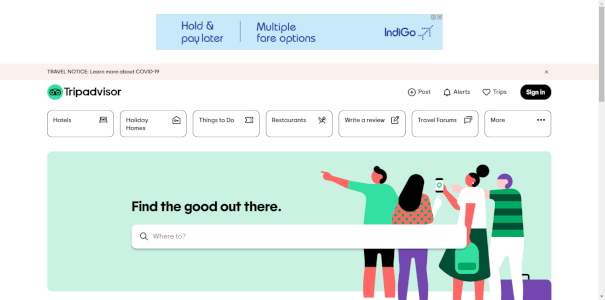The image displays a TripAdvisor webpage with a predominantly white background, interspersed with various colored sections. Centered at the top is a light blue rectangular banner divided into three segments. The left segment reads "Hold and Pay Later" in blue letters, followed by a horizontal line, and the middle segment states "Multiple Fare Options" also in blue. The right segment features "INDIGO" along with an airplane icon, and an "X" button to close the banner.

Beneath this is a thin, light pink band stretching across the screen, displaying a travel notice about COVID-19 and an arrow on the right end to dismiss the message.

Further down, the TripAdvisor logo appears in black on the left, featuring iconic owl eyes. To the right are several icons reading "Trips" (unclear text), "Alerts," "Tips," and a sign-in option within an oval button.

Below the primary sections, a series of smaller horizontal rectangles with light gray borders represent different site options: "Hotels," "Holiday Homes," "Things to Do," "Restaurants," "Write a Review," and "Travel Forums."

Towards the bottom of the image, there is a lighter blue section containing a search bar with the text "Find the Good Out There." Adjacent to the search bar, digital artwork depicts four people, likely travelers (two men and two women), standing with luggage. One person holds a backpack, while another appears to be looking at a cell phone.